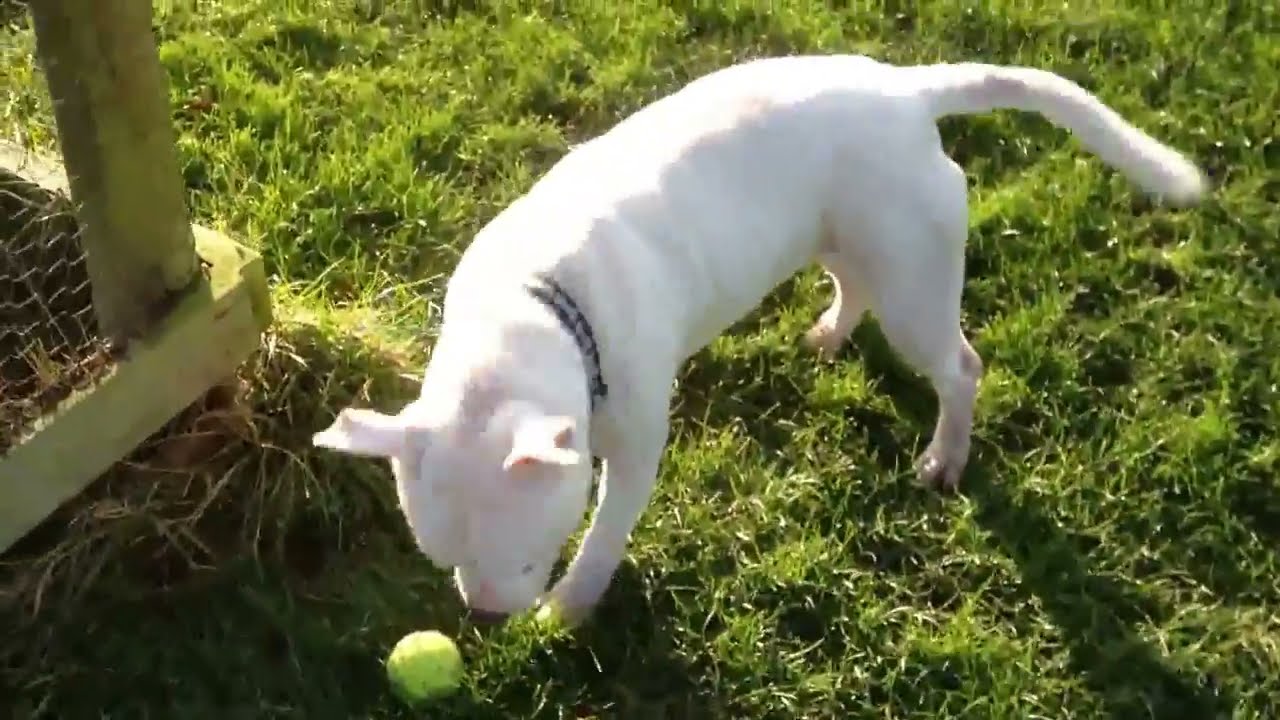In this outdoor image dominated by a grassy background, a medium-sized, all-white dog, likely a pit bull, takes center stage. The dog, standing sideways in the middle of the picture, has its head down, seemingly focused on a bright yellow tennis ball lying at its feet. The dog wears a black collar adorned with little white bone patterns. On the left side of the picture, partially visible, is an outdoor structure resembling either a cage or a chicken coop, made of wood and metal chicken wire. The vivid sunlight highlights the grass, indicating it could be midday or a time when the sun is particularly bright. The overall setting is a serene backyard scene with no people or text, and the palette includes green, white, black, brown, and hints of pink and tan.